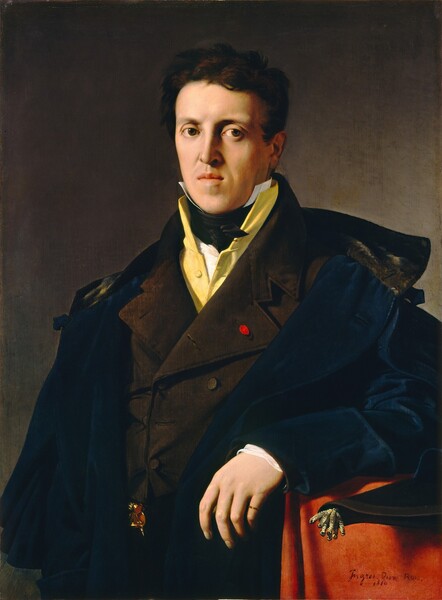The image depicts a surly, stern-looking Caucasian male with short black hair and brown eyes, dressed in a traditional general's uniform. He stands in a classic, commanding pose reminiscent of Napoleon Bonaparte, though the identity noted at the bottom remains indecipherable. The general's attire includes a dark blue overcoat draped over a brown coat, beneath which peeks a yellow shirt with a tall collar, partially obscured by a black neckerchief. A white shirt with a tall collar is layered underneath, creating a detailed and formal ensemble. His left hand rests on an orange-red tablecloth-covered table, while the right hand is out of frame. The background transitions from a dark blue or gray on the upper left to a lighter gray on the right. A peculiar protrusion near his arm, resembling a lizard or bird limb, adds an unusual element to the painting, which overall presents a vivid image of historical military dignity.